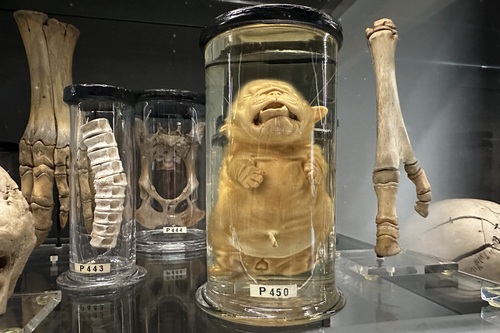The image depicts a meticulously arranged display likely from a scientific lab or a museum exhibit. Central to the display are several clear jars with black lids, each containing preserved specimens labeled with codes such as P450, P403, P443, and P444. The foremost jar houses a peculiar yellowish specimen resembling a juvenile creature; it has tiny arms and fingers, a slightly open mouth exposing two small fangs, somewhat reminiscent of a "cat troll" or a "large, obese kitten." Another jar in the background is labeled P403 and contains what appears to be a spinal column, while a third jar labeled P444 harbors an object that might be a pelvic bone or similar in shape to a bat. The scene includes bone fragments and other skeletal structures resting on the glass table, contributing to the overall eerie and intriguing ambiance. The backdrop is dark blue, enhancing the display's focus within a possible glass case, suggesting an exhibit designed to be viewed but not touched by the public.